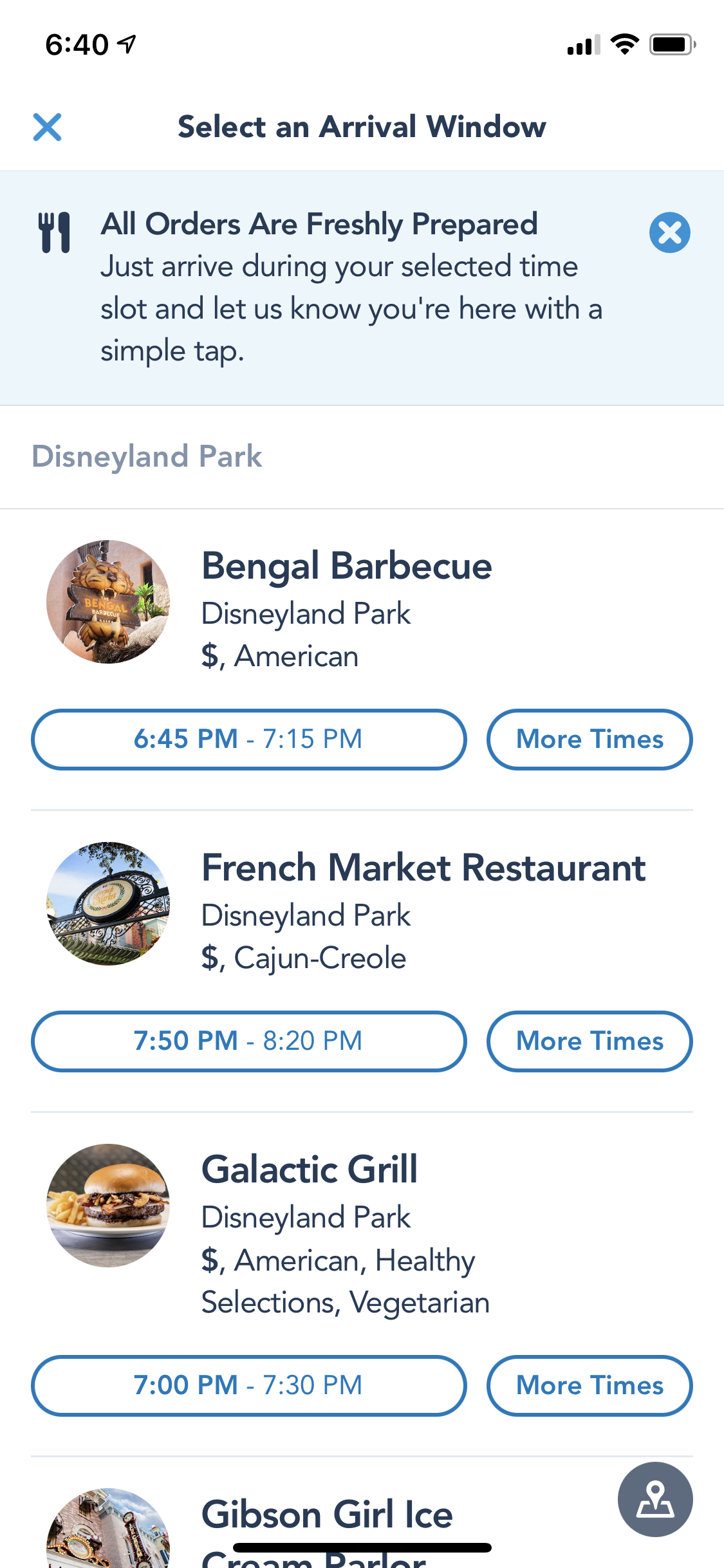This image captures a smartphone screen displaying a Disneyland dining reservation interface. At the very top, the status bar shows the time as 6:40, alongside an airplane mode icon, signal bars, a Wi-Fi symbol, and a nearly full battery indicator, approximately at 95%.

Beneath the status bar, a header contains a blue 'X' next to the prompt "Select an Arrival Window." Below this, a message accompanied by fork and knife icons states: "All orders are freshly prepared. Just arrive during your selected time slot and let us know you're here with a simple tap."

Following this, the screen lists dining options:
1. **Disneyland Park - Bengal Barbecue**
   - Cuisine: American
   - Price: $
   - Time slots available: 6:45 PM - 7:15 PM
   - A button labeled "More Times" is present for additional availability.

2. **Disneyland Park - French Market Restaurant**
   - Cuisine: Cajun, Creole
   - Price: $
   - Time slots available: 7:50 PM - 8:20 PM
   - Another "More Times" button is available for more options.

Further down, additional dining options such as the Galactic Grill and Gibson Girl Ice Cream Parlor are mentioned, suggesting similar selection mechanisms for arrival windows and additional times.